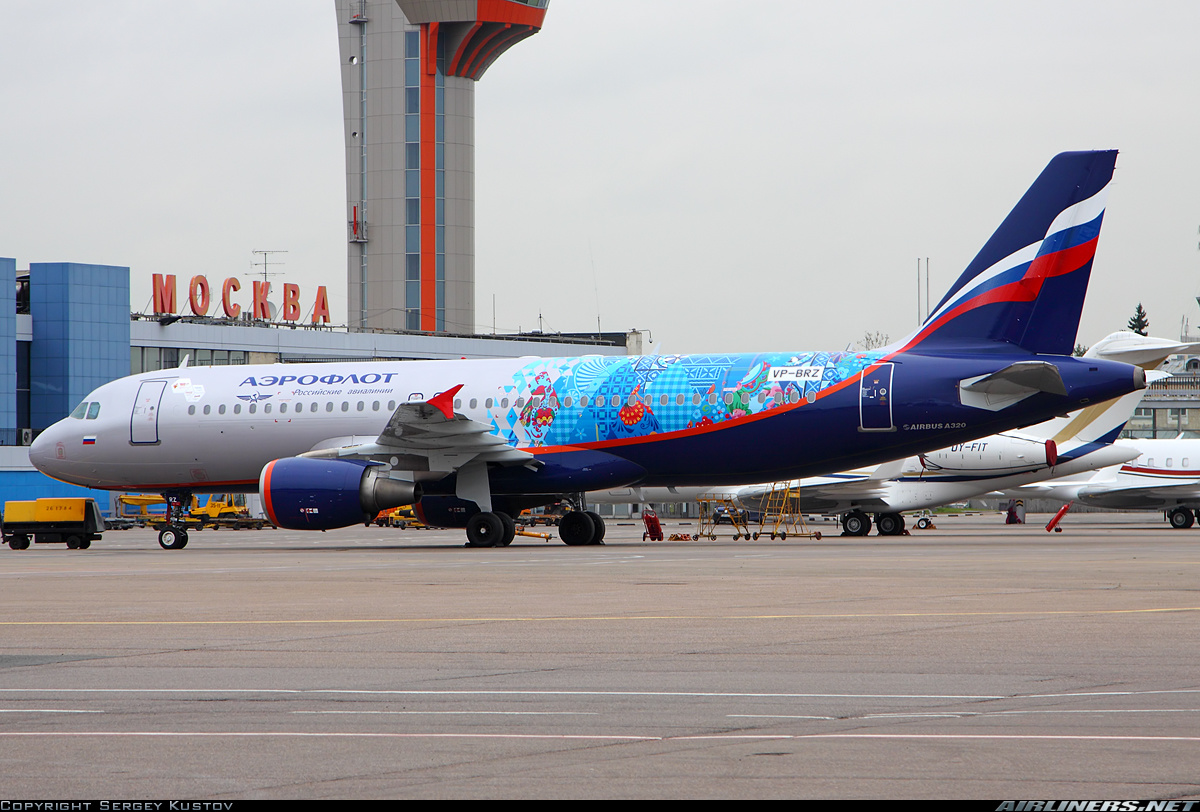This is a detailed daytime photograph taken at a Russian airport, showcasing a prominent silver and blue passenger airplane positioned centrally on the tarmac, facing left. The airport terminal in the background displays the sign "Москва" (Moscow) in Cyrillic, beneath a tall concrete air traffic control tower adorned with bright cherry red and blue accents. The airplane, possibly an Aeroflot flight, features a distinctive dark blue tail and engine housing. A ribbon mirroring the colors of the Russian flag—white, blue, and red—adorns the tail, along with a colorful design that appears to be a world map incorporating reds, electric blues, light blues, greens, and pinks. Ground crew members are visible below the aircraft, handling luggage among numerous taxi-yellow service carts and ladders. Several other planes, primarily white and minimally decorated, are partially visible in the background, obscured by the central aircraft. A signature in the bottom left reads "copyright Yersi Kustov," and the bottom right is marked "airliners.net."